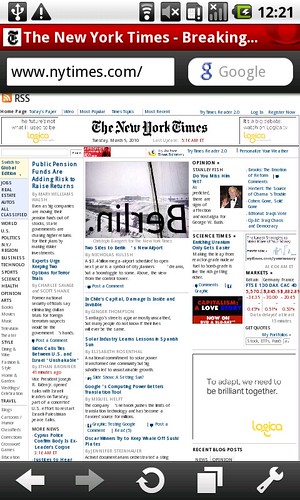A screenshot of the device screen displays the New York Times website, with various icons and notifications visible. At the top, there are navigation options including back, forward, and refresh buttons. The screen also shows tabs, settings, USB debugging icon, a triangle with an exclamation mark, Wi-Fi signal, silent mode icon, a gas pump icon, a calculator, and the battery status indicator. The current time reads 12:21 PM. The text "You are good" is also visible on the image.